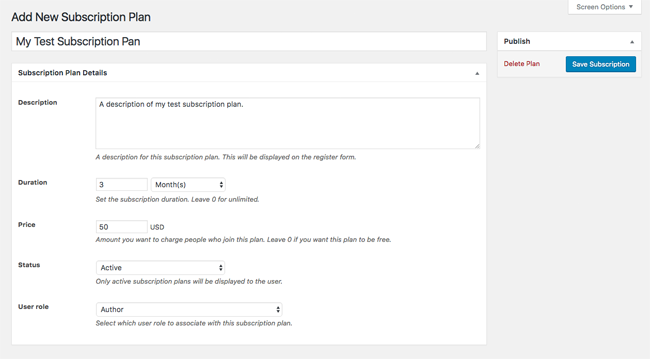The image depicts a webpage or a pop-up window with the title "Add New Subscription Plan" prominently displayed at the top of a light gray background. To the right of this title, a box extends from the top right-hand corner of the page, labeled "Screen Options" in gray font. The main title and the majority of the text on the page are in black font, with accented text in red and white within a box on the right side.

Immediately below the main title, there is a white input box containing the text "My Test Subscription Plan" in black font. Beneath this, another box is titled "Subscription Plan Details." This section includes various fields such as "Description," "Duration," "Price," "Status," and "User Role." Each of these fields allows for customization:
- "Description" for entering text details about the plan,
- "Duration" with options to specify in months, years, or days,
- "Price" in USD,
- "Status" having selectable options like active or inactive,
- "User Role" which can also be customized.

To the right of these descriptive fields, there is a functional box containing actionable options. It includes a "Publish" button, a red link labeled "Delete Plan," and a blue button with white text reading "Save Subscription."